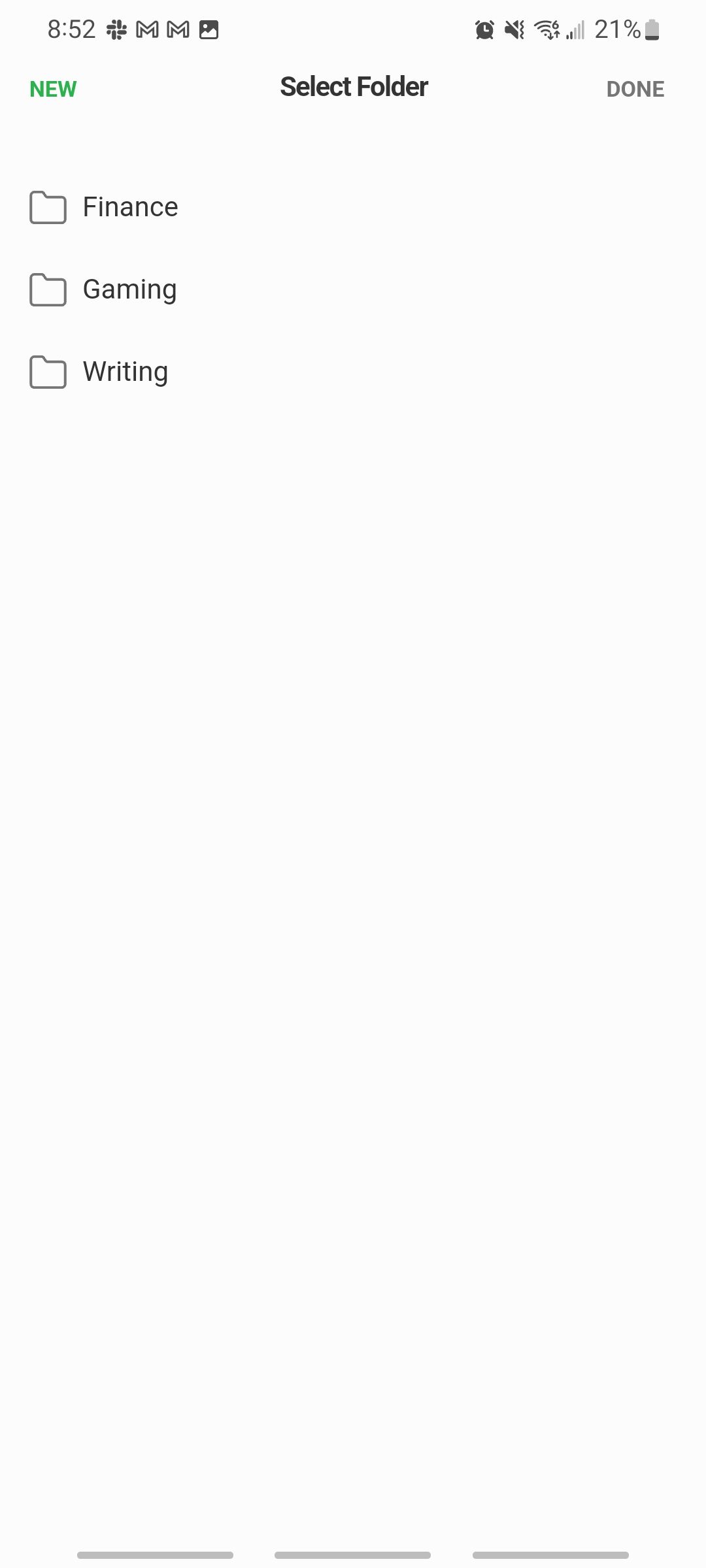The image displays a smartphone screen at 8:52 AM, featuring various icons and a clear user interface. At the top, there's a flower symbol, followed by Gmail, Photos, Clock, and a speaker icon indicating muted sound. The Wi-Fi icon shows full signal strength, while the cell signal is not at full strength, and the battery is at 21%. There's green text labeled "New," black text saying "Exact Folder," and gray text reading "Done." Three folders are visible: "Finance" at the top left, "Gaming," and "Writing." The background shows the "Writing" folder open, while a gray line spans the bottom, accompanied by three smaller gray lines indicating additional pages or sections. The overall layout confirms it's a typical smartphone interface, complete with organized folders and essential app icons.